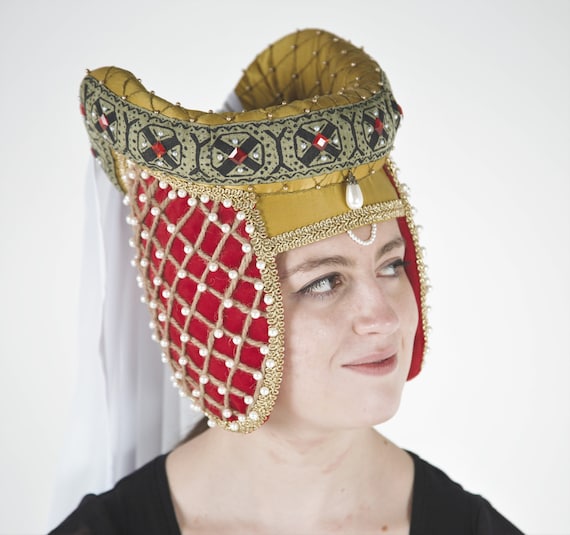The image features a young girl set against a light gray background, adorned with an intricate piece of headgear resembling that of a princess or queen. The headpiece is crafted from cloth and shaped into a rounded silhouette, showcasing a brownish-yellow hue. Overlaying the cloth, a delicate netting adorned with small gold beads adds a touch of elegance. A prominent band, detailed with red X's and studded with various jewels, spans across the headpiece. Centrally positioned, a significant drop pearl hangs, accentuated by a loop of smaller pearls resting at the forehead. The netting continues behind this arrangement, maintaining the brownish-yellow theme. The headpiece further extends to include two large, red ear pieces, which are similarly overlaid with netting and decorated with white jewels, completing the regal attire.